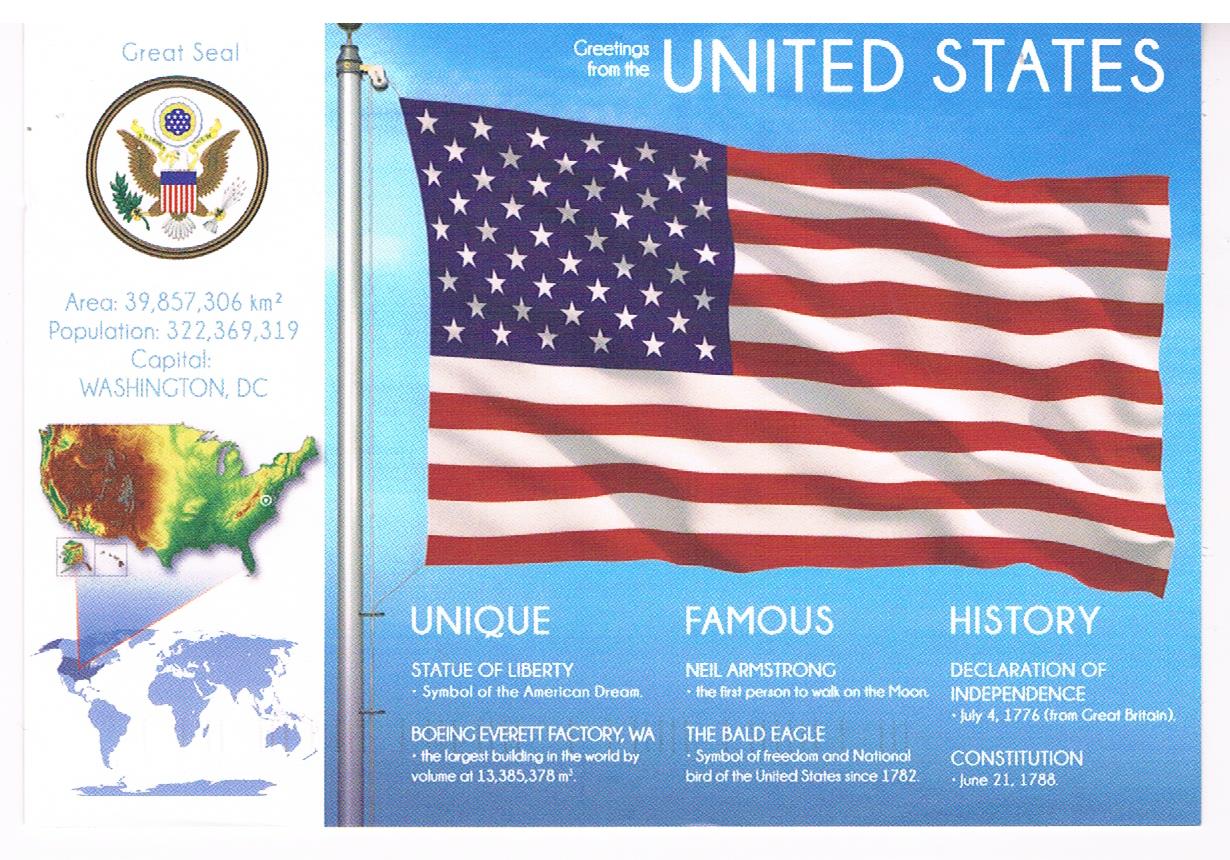This image appears to be a scanned page from an old magazine ad, likely from the 80s or 90s, and features a detailed patriotic theme centered around the United States. Dominating the center is an American flag on a cylindrical pole, waving against a blue sky background. Above the flag, white lettering reads, "Greetings from the United States." Below, the image divides information into three white-lettered categories: "Unique" (highlighting the Statue of Liberty and the Boeing Everett Factory in Washington), "Famous" (featuring Neil Armstrong and the bald eagle), and "History" (covering the Declaration of Independence and the Constitution). To the left side, it displays the Great Seal of the United States, with the bald eagle clutching arrows in one talon and an olive branch in the other. Beneath the seal, it lists the country’s area as 39,157,000 square kilometers, population as 322,369,319, and the capital as Washington, D.C. A map of the United States in green, yellow, and red is shown below this information, followed by an expanded view to place North America within the global context. The poster encapsulates iconic symbols and historical elements of American culture, set against a vivid and nostalgic backdrop.